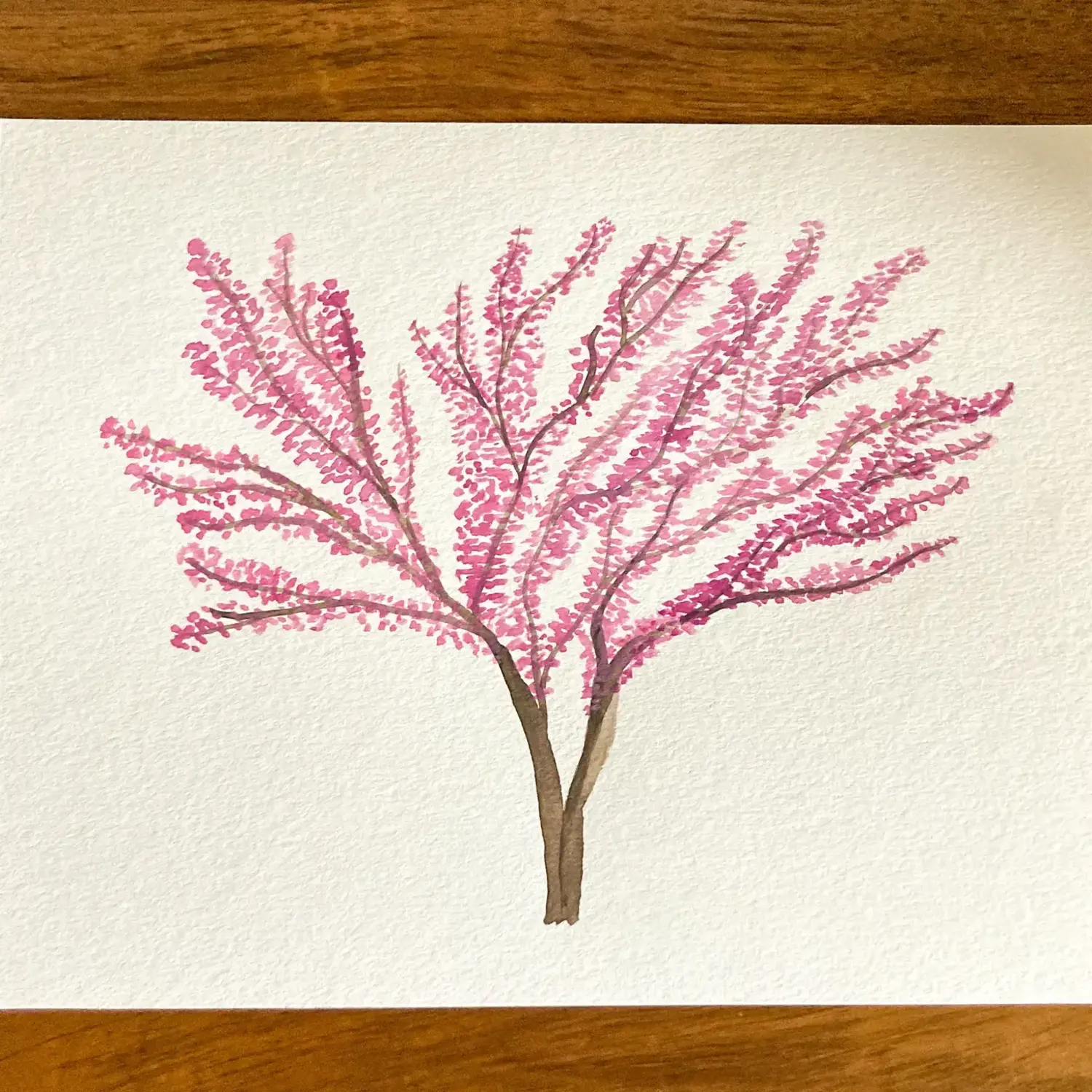This photograph captures a detailed watercolor painting of a cherry blossom tree, set on a creamy, textured, rectangular canvas that almost resembles thick, handmade paper. The painting features a slender brown trunk that splits into two, gracefully extending upward and outward into a web of branches adorned with various pink hues of blossoms. The blossoms are created with small, delicate brushstrokes, giving the impression of abundant cherry blossoms in both lighter and darker shades of pink. The canvas is placed on a glossy, medium brown oak table, with its horizontal wood grain adding a contrasting textured backdrop to the simplicity of the artwork.